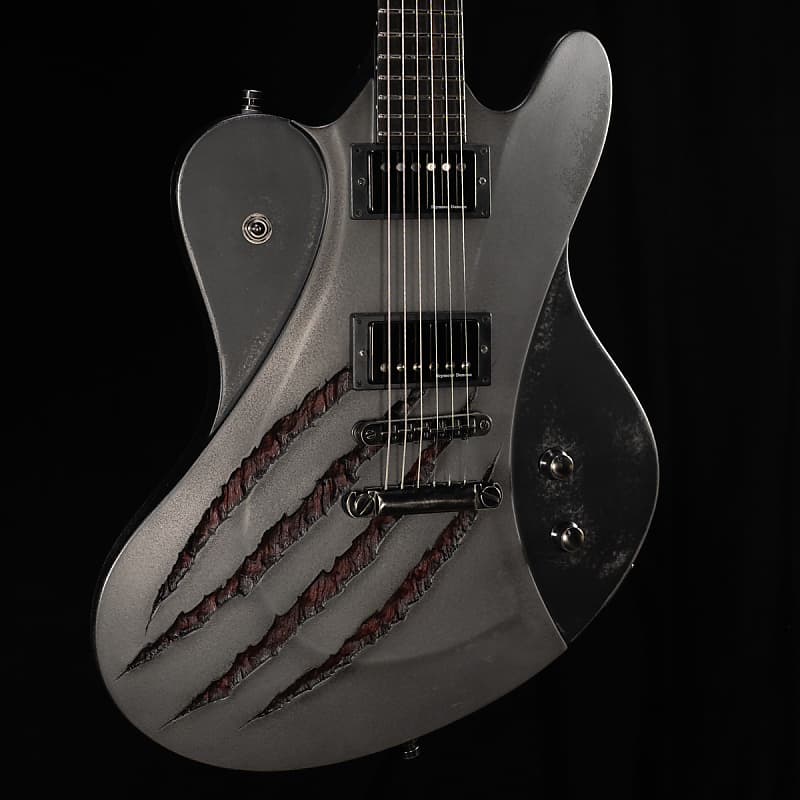This stylized black-and-white photograph showcases an electric guitar set against a jet black background. The guitar's body features a contrasting design, with the central area being a light gray or silver color and the outer edges in black. The upper-left and lower-right sections of the instrument's body are particularly noteworthy; the upper-left section is a dark gray, almost black teardrop shape with a music jack, and the lower-right has black with silver dials and a button. Silver strings extend from a metal bar at the base, disappearing at the top where the fretboard, which is also black, begins.

Prominently displayed on the light gray central part of the guitar are four dramatic, claw-like scratch marks, suggesting an encounter with a wild animal. These slashes are jagged and intense, cutting through the surface and revealing a dark, possibly reddish interior. The guitar does not include the traditional round soundhole; instead, it features two horizontally rectangular openings outlined in dark gray metal. These openings are positioned near the center and slightly lower on the body, contributing to the guitar's unique, visually striking design.